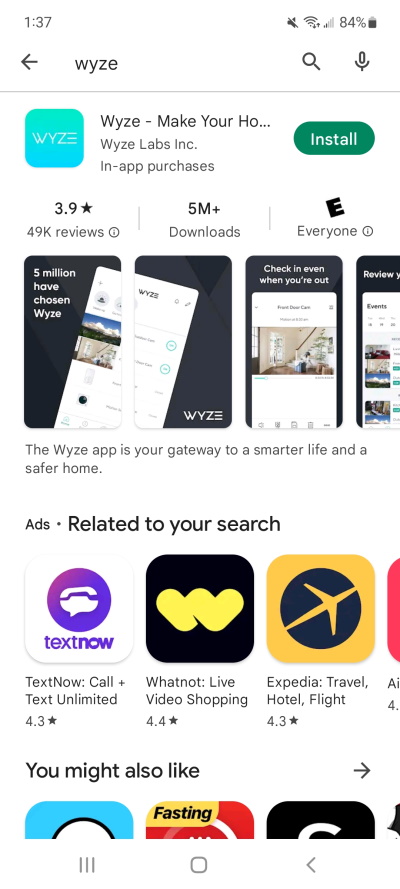The screenshot displays the Google Play Store page for the "WiZ" app, a smart lighting control application. In the top part of the screenshot, standard cell phone icons are visible on the upper left and right-hand sides, indicating battery life, signal strength, and other status symbols.

The highlighted app, "WiZ," is prominently displayed just beneath these icons. The app's interface showcases a green "Install" button, signifying that it is ready for download. Additional information about the app includes over five million downloads and an average rating of 3.9 stars from approximately 49,000 user reviews. The app is rated suitable for all age groups.

Below this information, four preview images of the application are arranged horizontally, providing visual insight into the app's interface and functionality. A brief description follows these images, elaborating on how the WiZ app enables users to control various smart lighting products, suggesting its utility for any smart home enthusiast.